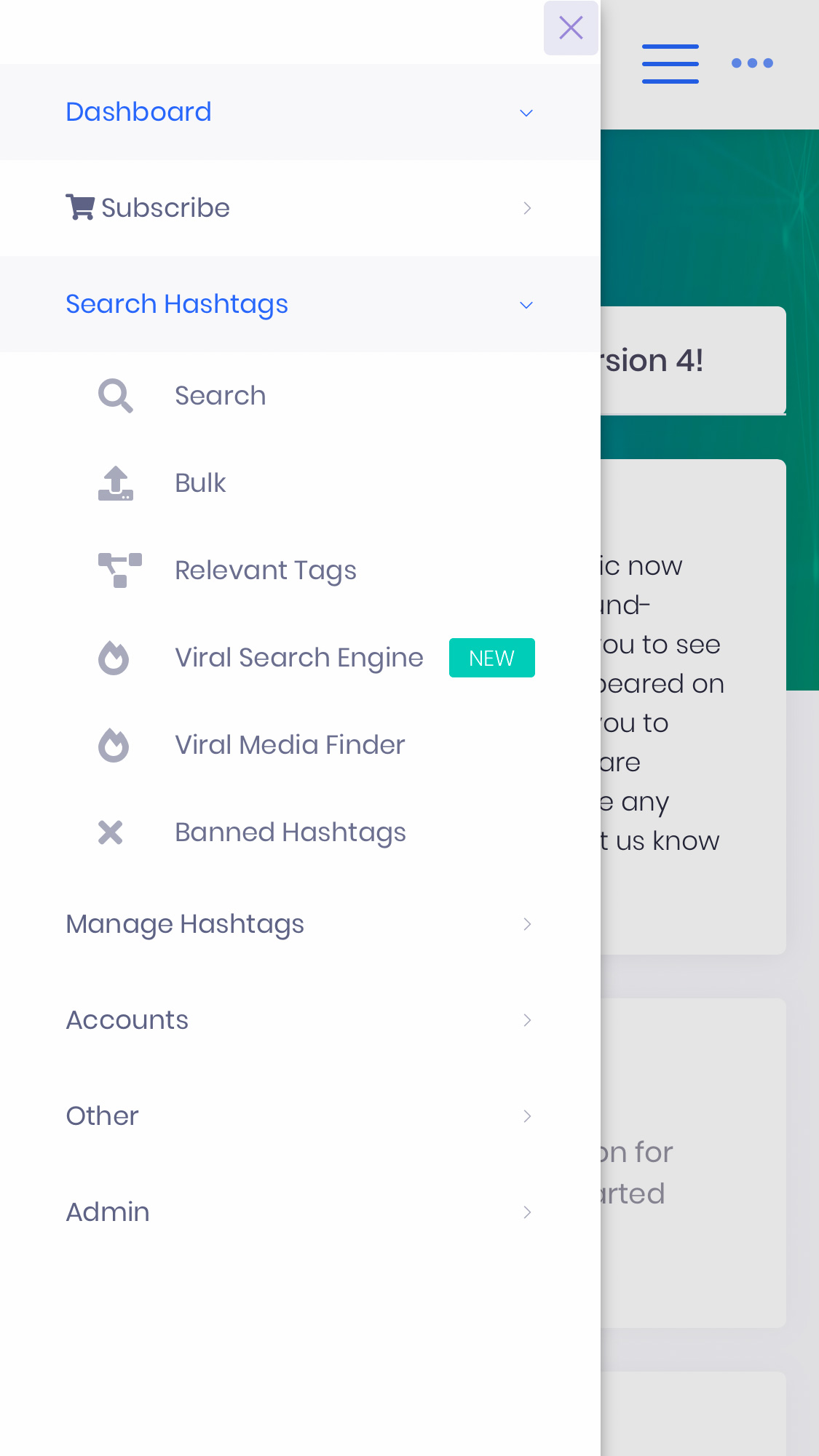The image is a screenshot of a phone screen, prominently featuring a pop-up window that obscures two-thirds of the left side of the display. Noticeably, typical phone status indicators like battery life are absent from view. 

The large pop-up window has an "X" at the top-right corner for closing it. Below this, the window contains several interactive elements. At the top, there is a gray rectangular drop-down menu labeled "Dashboard." Directly beneath this, there's a white button labeled "Subscribe" with a side arrow indicator, followed by a gray rectangle that reads "Search Hashtags" in blue. This blue text suggests an active or open drop-down menu.

Further down, the window displays several icons paired with text that provide different functionalities. These include "Search," "Bulk," "Relevant Tags," and "Viral Search Engine," the latter of which is tagged with a green "New" button. Additional options include "Viral Media Finder" and "Banned Hashtags." 

Towards the bottom, several gray rectangles contain labels with side arrows, including "Manage Hashtags," "Accounts," "Other," and "Administration," indicating that these sections can be expanded for more options.

The backdrop of the pop-up is a teal-green screen with partially obscured text at the top, which appears to reference "session four" followed by an exclamation point. The remaining content of the background is largely unreadable due to the overlay of the pop-up window.